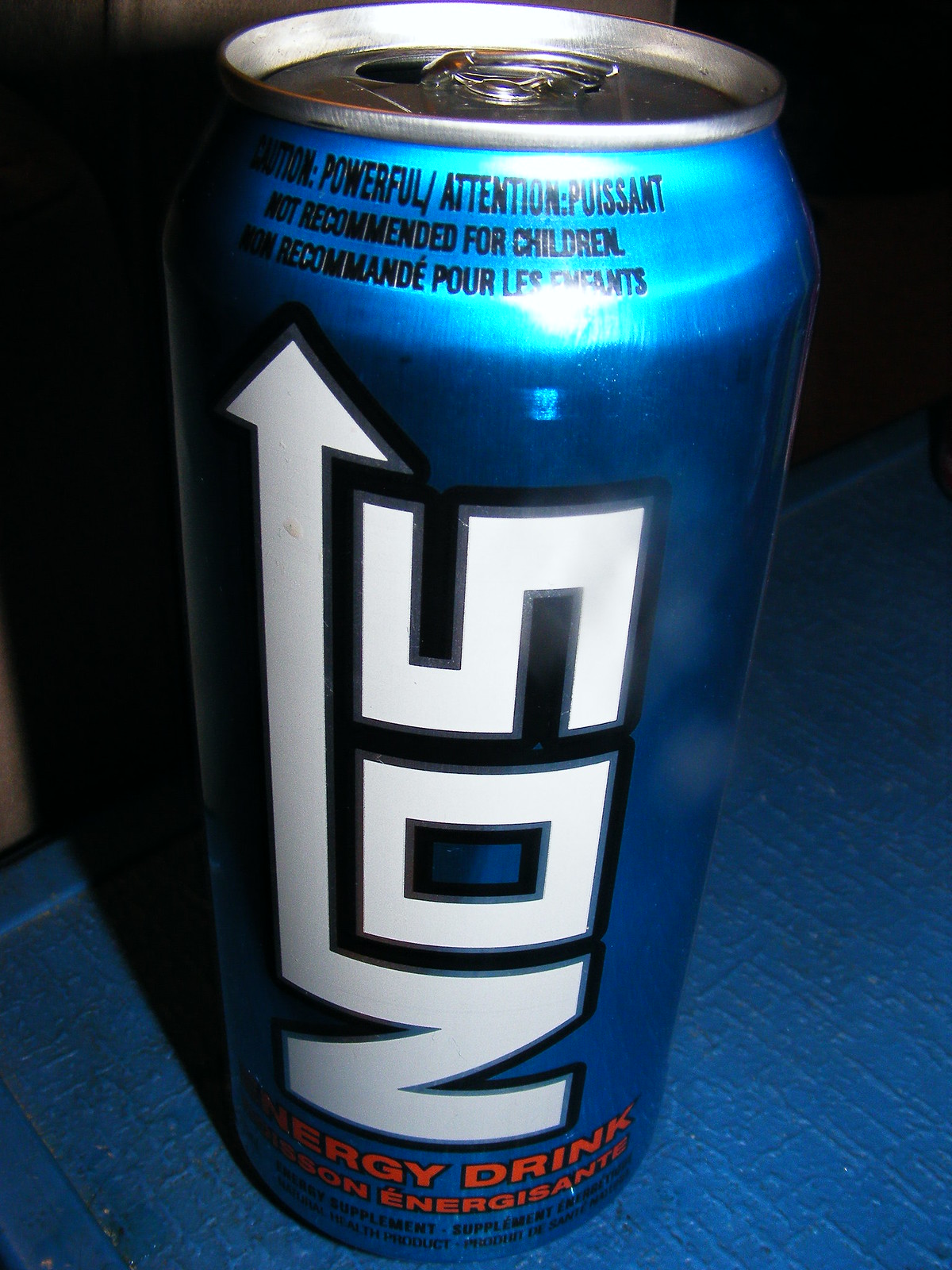This color photograph features a close-up of a bright blue NOS energy drink can, which is the size of a typical soda can and sits atop an indistinguishable blue surface, likely a table or counter. The can's pull tab has been opened, though it appears oddly distorted, as if melted, raising suspicions of the image being artificially generated. Prominent on the can is the NOS logo, a white text outlined in black with an arrow extending from the "N" and crossing over the rest of the letters. Below this, orange text indicates "Energy Drink." There are multiple cautionary and promotional phrases on the can, such as "Caution, Powerful, Attention," and warnings in both English and French, stating "Not recommended for children" and "Non-recommandé pour les enfants." The reflective surface of the can catches the flash from the camera, and despite some text being partially out of view around the curvature of the can, the intricate details and reflections add to the image's striking appearance.